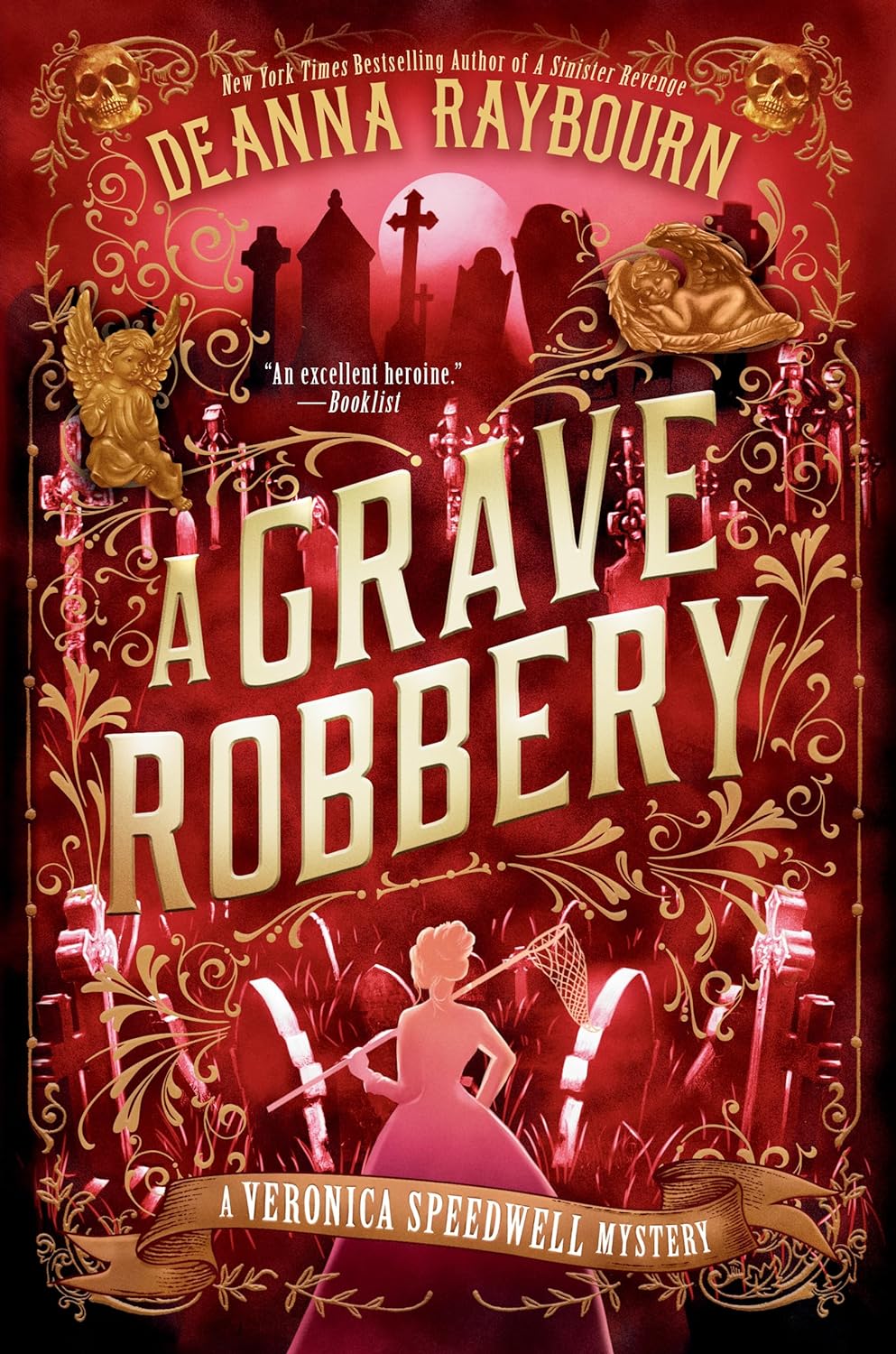The book cover is a detailed color illustration with a dark red background dominated by a cemetery scene silhouetted at the top, featuring a rising white moon and a pink sky. At the very top, in small gold lettering, it states "New York Times best-selling author of A Sinister Revenge." Below this, in larger gold type, is the author's name, Deanna Raybourn. Flanking this text on both sides are gold, cherubic cupids. A central arc in gold type highlights the book's title, "A Grave Robbery," with reflective gold letters. Just above the title, a review in white text reads, "An excellent heroine," attributed to Booklist. The bottom portion of the cover features a pink silhouette of a woman in a long dress, holding a net over her shoulder. Beneath her, a gold banner declares the book as "A Veronica Speedwell Mystery." The composition presents a striking and eerie yet sophisticated theme that fits the novel's mysterious tone.